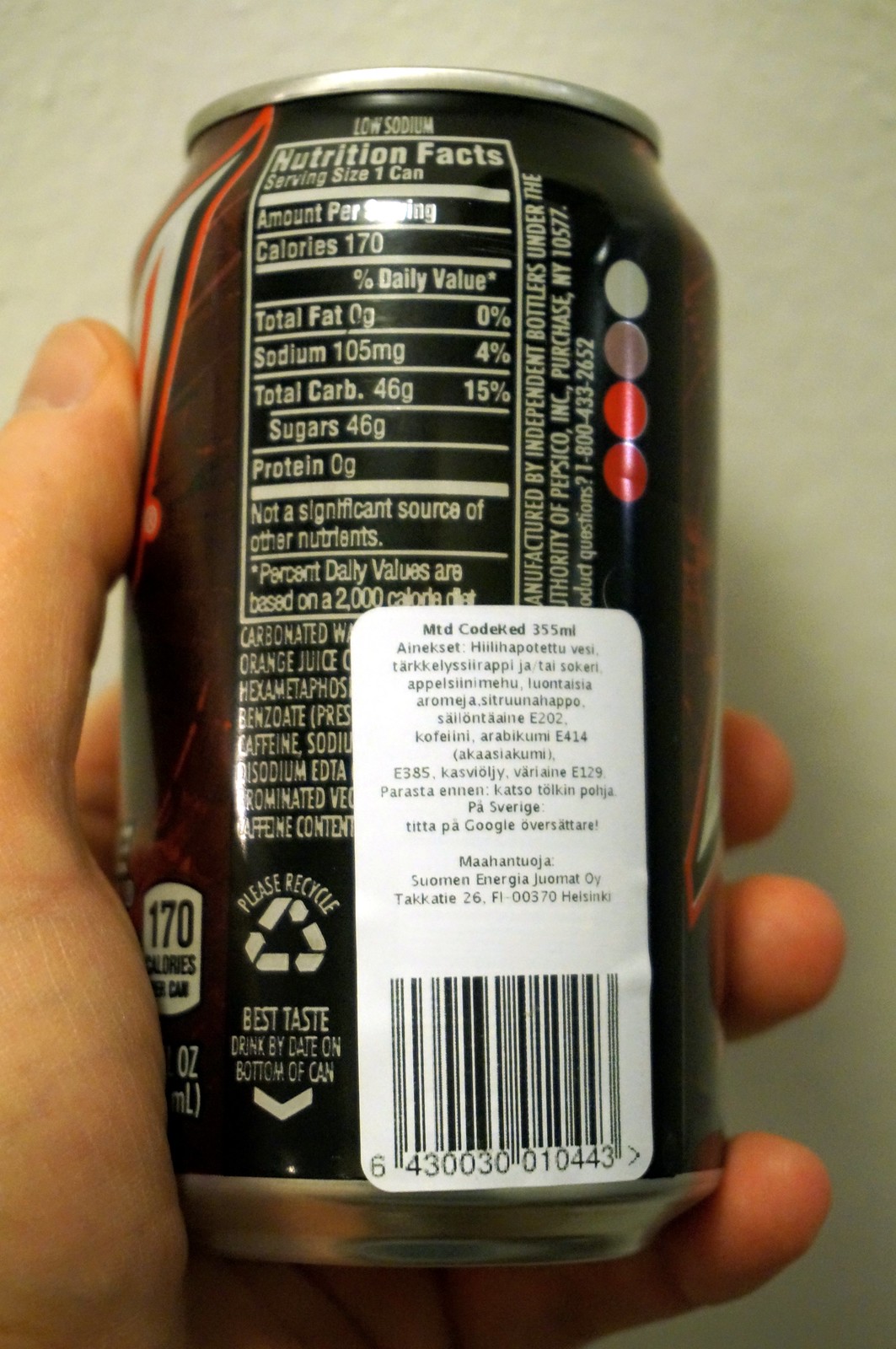In the image, a Caucasian person is holding up a black can of Mountain Dew, likely Mountain Dew Code Red, in their left hand. The hand positions the can so that the nutrition facts label faces the camera, with their thumb on the left side and fingers wrapping around the right. The nutrition details visible on the can include: 170 calories per serving, 0 grams of total fat, 105 milligrams of sodium (4% of the daily value), 46 grams of total carbohydrates (15% of the daily value), 46 grams of sugars, and 0 grams of protein, with a note that it is not a significant source of other nutrients. The label further indicates that daily value percentages are based on a 2,000 calorie diet. Below the nutrition facts, the ingredients are listed, but partly obscured by a white sticker featuring black text in a foreign language and a barcode. Symbols at the bottom indicate the can is recyclable and that it maintains the best taste by the date on the bottom of the can. A light shine creates some reflection on the can, with a shadow against the gray wall background, which occupies the majority of the photograph.